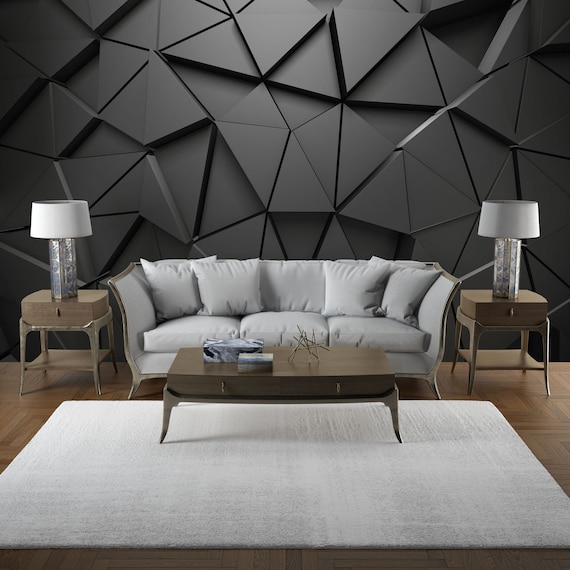This image depicts a modern living room setting. The centerpiece is a light gray, three-seater sofa adorned with four small matching off-white pillows, placed symmetrically with two on each side. Flanking the sofa are two light wooden end tables, both topped with identical silver lamps with off-white rectangular shades. In front of the sofa is a matching wooden coffee table, upon which rests an art piece resembling clustered sticks and a few boxes. Beneath the coffee table lies a neat off-white rectangular rug. The floor, extending the length of the image, is made of medium brown hardwood. The striking feature of the background is a dark gray, three-dimensional wall, detailed with a continuous pattern of various triangular shapes, creating a dynamic, textured effect.